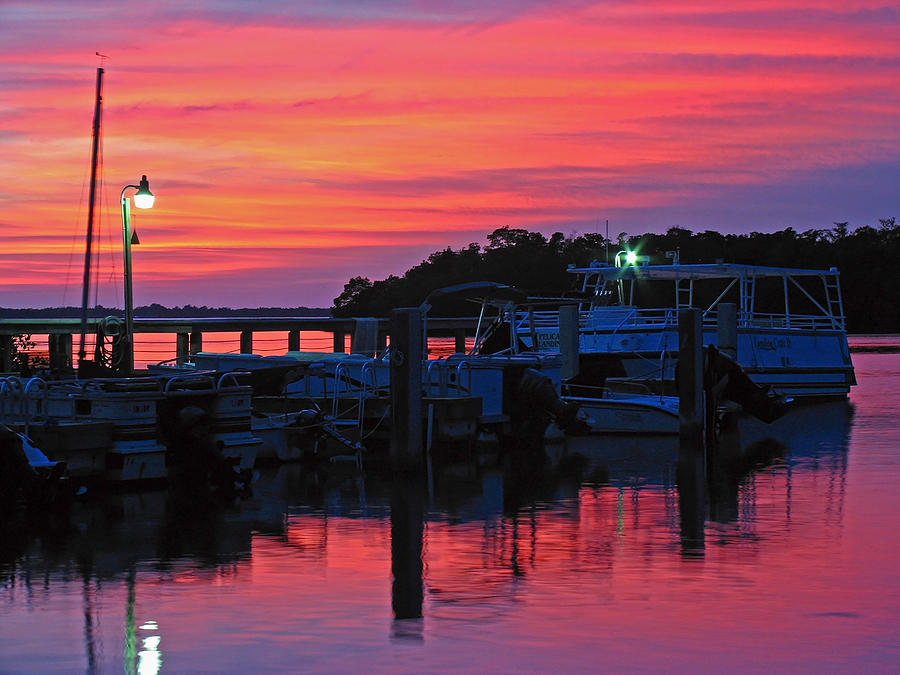This high-quality image captures a breathtaking sunset at a serene boat marina, where the sky transitions through mesmerizing hues of orange, pink, purple, and blue. The vibrant colors reflect off the calm, still waters of the lake, imparting a pinkish-purplish glow. A wooden dock stretches into the lake, punctuated with slots for multiple boats; there are at least six boats docked. A variety of vessels are moored here, including a pontoon boat with a canopy and a light on, a couple of fishing boats, and a larger pontoon boat at the end of the dock. A green lantern-style floodlight illuminates the wooden walkway running down the center of the dock. The scene is enhanced by an island silhouetted with trees in the middle distance. Wooden poles rise from the water, adding to the peaceful ambiance of this picturesque marina.